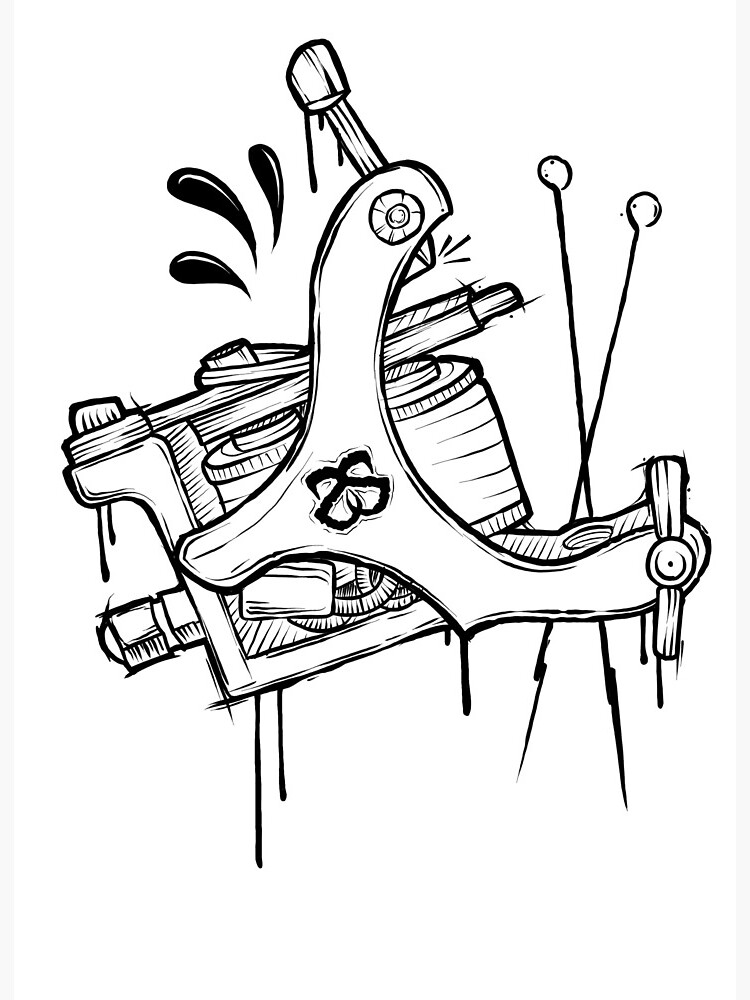This black-and-white illustration depicts a tattoo machine rendered as if meticulously carved from wood. Dominating the image is a C-shaped mainframe, adorned with a distinctive logo comprised of a backwards S mirrored by a regular S, both in bold black. Extending from this main body is an intricate array of components, including three cylindrical elements entwined with horizontal bands or strings, and situated above a set of three gear-like structures. An L-shaped framework supports the rear, linked to the cylinders by additional bands. The top of the illustration shows three black, upside-down, teardrop-shaped marks reminiscent of ink splatters. At the forefront of the C-shaped frame, a knob with vertical and horizontal handles is visible, accompanying two crossed needles with loops at their tips on the right side. The illustration, though monochromatic, suggests a textured, hand-carved wooden appearance through its intricate details and irregular markings.